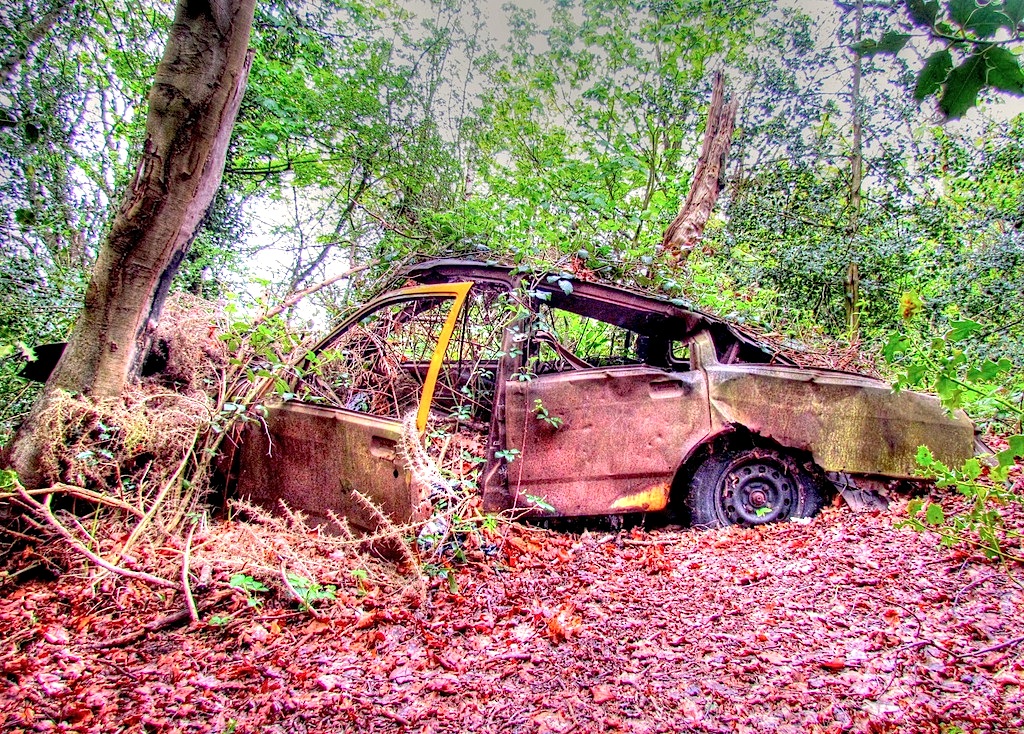The image depicts a heavily decayed and decrepit car, possibly a hatchback, that appears to have been abandoned for decades in a dense forest setting. The car is severely damaged, with the roof crushed in, the back end bashed, and one door detached and hanging open. A mixture of red and brown leaves, suggesting it's autumn, blanket the ground and have crept inside the vehicle. The forest surrounding the car is lush with green trees and stumps, and the sky above is cloudy. The car's once-yellow paint is largely eroded, blending into the natural surroundings. The car is positioned sideways, obscuring the make and model, and it is enveloped by vegetation, with plants growing inside and around it, seemingly becoming part of the forest itself. No people are visible, emphasizing the car's long-forgotten solitude in the woodland.